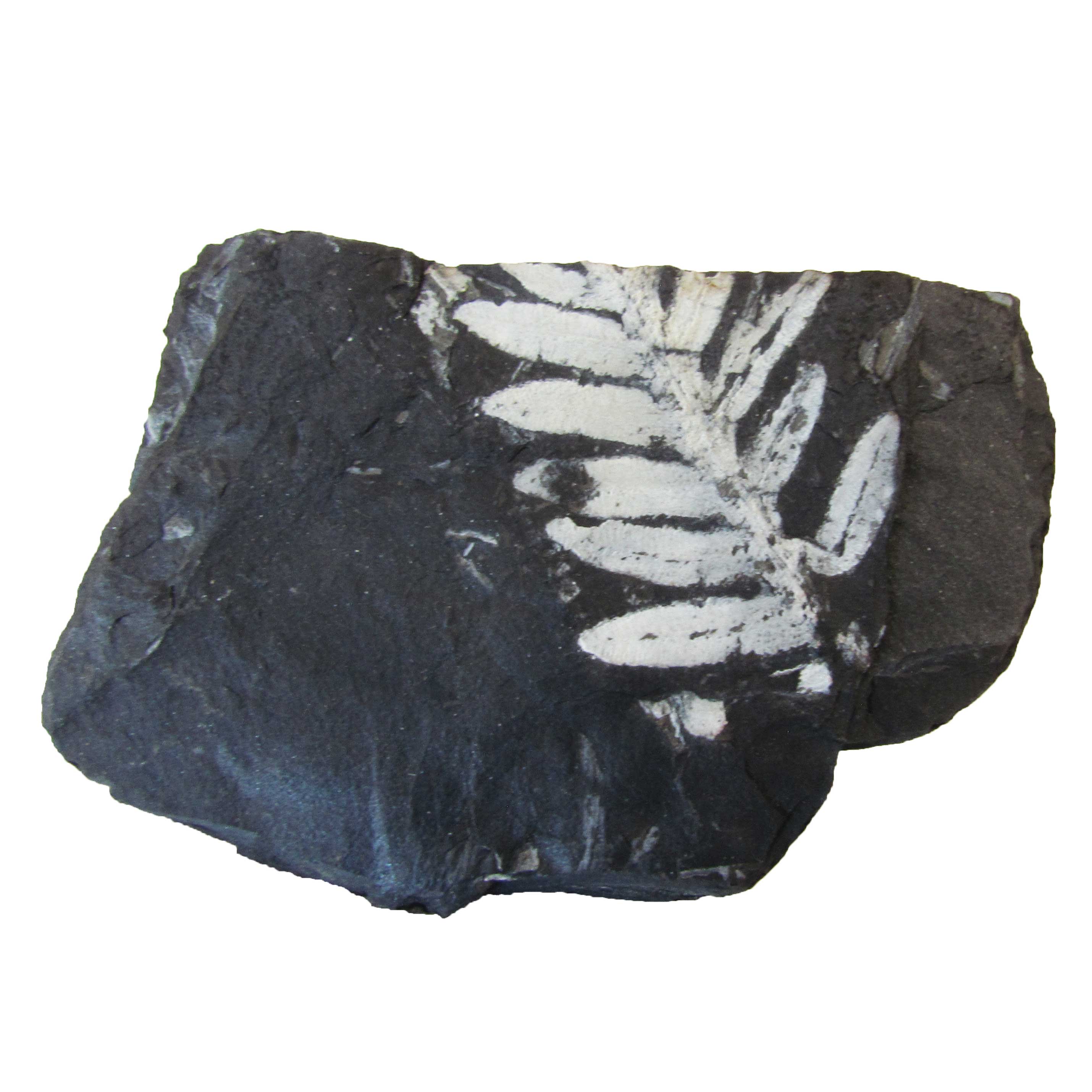The image depicts a piece of black rock, possibly basalt or flint, with a shiny, smooth surface that is flatter on the top and more irregular and rounded on the right and bottom. The background of the image is completely white, emphasizing the dark rock. Situated on the rock is a white imprint or painting of a leaf, starting from the middle top of the rock and extending towards the lower right. The leaf has a prominent stem with pointed, mottled leaves on either side—around six on the left and five on the right. The imprint includes detailed lines that divide the leaves into distinct parts. The top part of the rock, along with the top section of the leaf imprint, appears slightly broken off, suggesting the rock might be an ancient artifact or a piece of sculpted art, potentially cut from a mountainside.